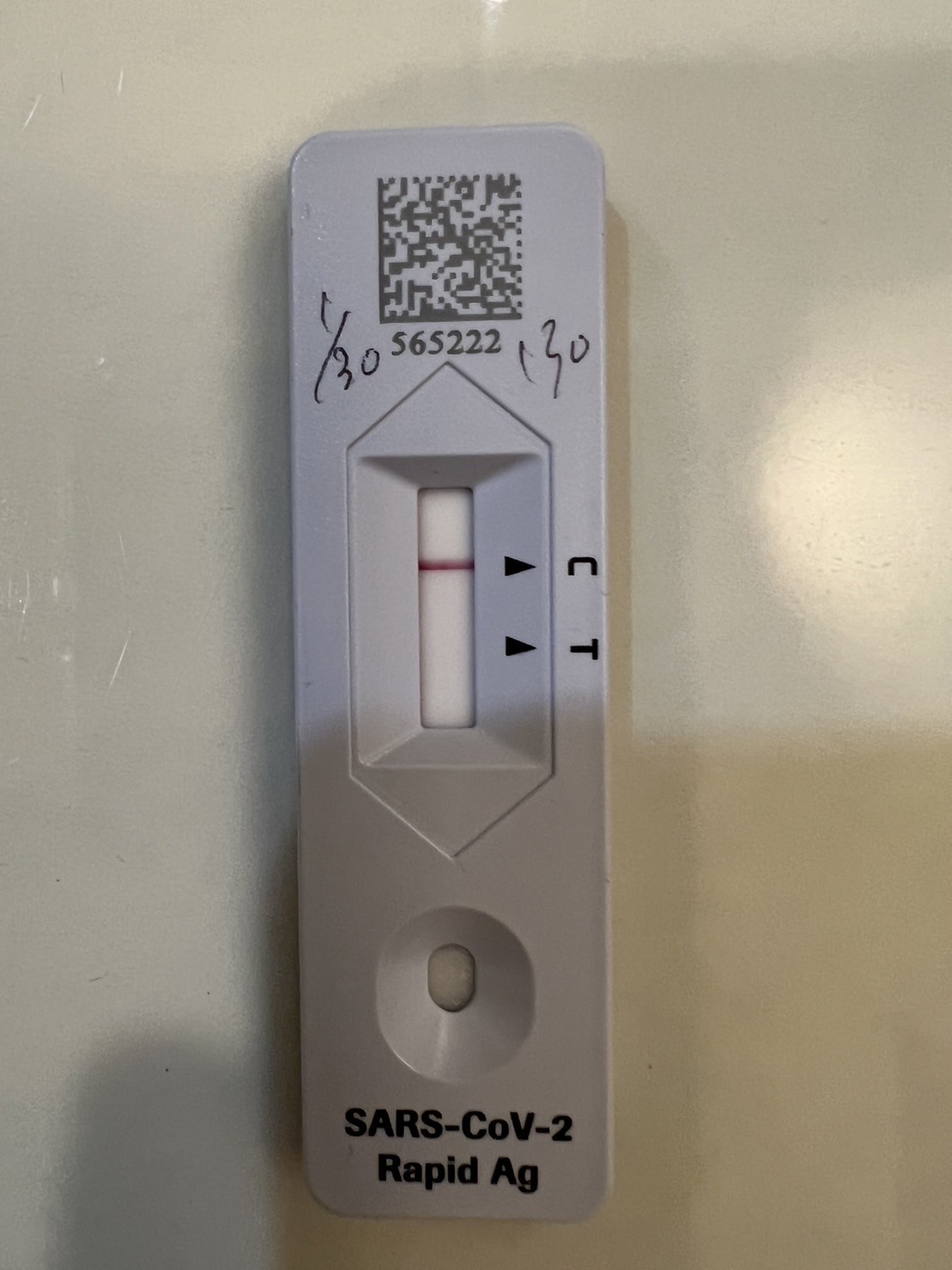The image depicts a gray, plastic device likely used for testing purposes, potentially for detecting radon, water quality, or more likely, as indicated by the label, the SARS-CoV-2 virus. The testing apparatus features two main regions labeled with capital letters "C" and "T". The top portion of the device may have a scannable code or patterned pixels, possibly for use with a smartphone, accompanied by a numeric code. 

In the middle of the device, a diamond-shaped indicator with a number "130" slopes inward towards a rectangular section. Here, a dark red or maroon line suggests this is the part of the device where the sample interacts with the indicator. Below this, there are two nested ovals: a smaller one set inside a slightly larger one, contributing to the overall concave shape of the plastic.

The bottom of the device is labeled "SARS-CoV-2 Rapid AG," clearly indicating that it is a rapid antigen test for detecting the COVID-19 virus. The testing device rests on a reflective white surface, though the exact nature of the surface is indeterminate. The numbers and letters on the device are black, providing high contrast against the gray plastic.